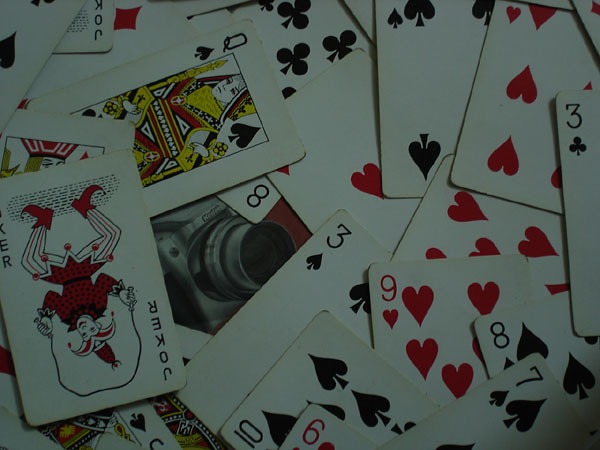In this close-up photograph, a chaotic pile of playing cards is scattered haphazardly across a maroon-colored tabletop, creating a striking, unorganized display. The cards, which include the Queen of Spades, Three of Spades, Nine of Hearts, Seven of Spades, Eight of Spades, Ten of Spades, and Three of Clubs, among various other visible suits, overlap each other in different directions. A Joker card stands out prominently, lying upside down atop the disarray. A small gap in the pile reveals the surface underneath, where a camera or camcorder in a silver or aluminum color can be glimpsed. The image captures the cards in a manner that makes them appear darkened, with none of them appearing to be a bright white.